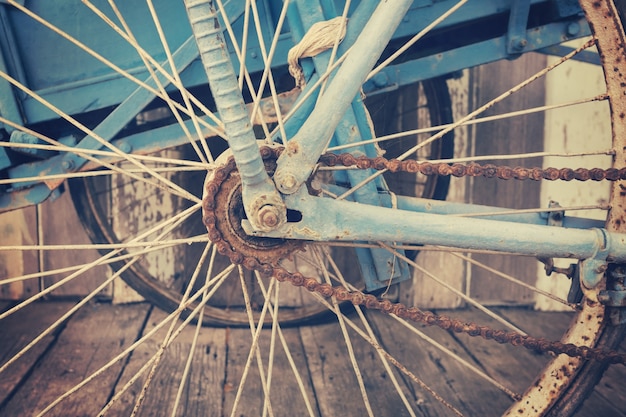This stylized photograph captures the central element of an older bicycle wheel with a rusted chain and gear. The focus is tightly on the white spokes, which exhibit a patina, highlighting the bicycle's age. The outer rim of the wheel also displays rust spots. The bicycle frame, painted in a light blue color, suggests further wear and tear, emphasizing the bike's vintage aesthetic. In the background, a wooden platform and slatted wood fence or possibly a shed provide context and set the scene, enhancing the rustic atmosphere. A secondary bicycle tire is visible, indicating the bike's ability to carry cargo, perhaps making it a single-speed utility or cargo bicycle. The entire composition of blues, whites, and rust tones evokes a nostalgic, timeworn charm.